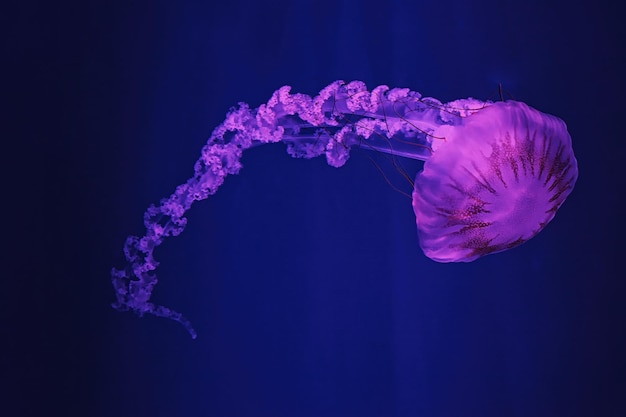This underwater photograph features a mesmerizing jellyfish, illuminated against a striking background. The background forms a horizontally rectangular canvas, transitioning from almost black at the edges to a deep royal blue in the center. The jellyfish is positioned on the right side of the image, exhibiting a mushroom-shaped head that is a captivating purplish-pink color, adorned with reddish-colored stripes radiating from the center to the edges. Below the jellyfish’s head, its long and windy trail extends towards the left, cascading downwards at the bottom-left of the frame. The trail shares the same pinkish-purple hue as the body, with some lighter and darker purple spots, and includes narrow red tentacles and a floral pattern-like appearance. The light shining down in the center illuminates the jellyfish, enhancing its ethereal beauty and creating a stark contrast with the dark, mysterious blues of the surrounding water.